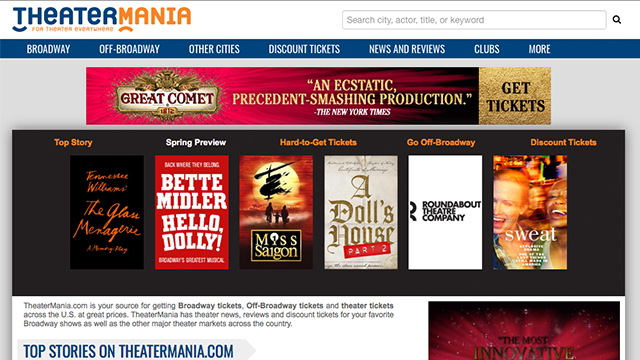This image is a screenshot of a website, specifically TheaterMania. The website's name is prominently featured at the top, with "Theater" in dark blue and "Mania" in orange. Below this, there are seven menu categories from left to right: Broadway, Off-Broadway, Other Cities, Discount Tickets, News and Reviews, Clubs, and More. Above these categories is a search bar.

Beneath the menu, there's an advertisement featuring a testimonial from The New York Times. The text "Great Comment and a Static Precedent Smashing Production" is displayed in gold text, followed by a white text attribution to The New York Times. To the right of the testimonial, there is a gold background with dark brown text that prompts users to "Get Tickets." The sides of the advertisement are bordered by a light gray background.

Further down the page, the user is presented with six movie covers and five categories. At the top are the categories, with the first, third, fourth, and fifth highlighted in orange, while the second category is in white. Below these categories is a very small gray paragraph of text. 

At the bottom left of the page, there is a "Top Stories on theatermania.com" section highlighted in blue. To the right, part of an image with a reddish-pink hue is visible, featuring a black background at the top. Additionally, light gray backgrounds frame parts of the left and right sides of the image.